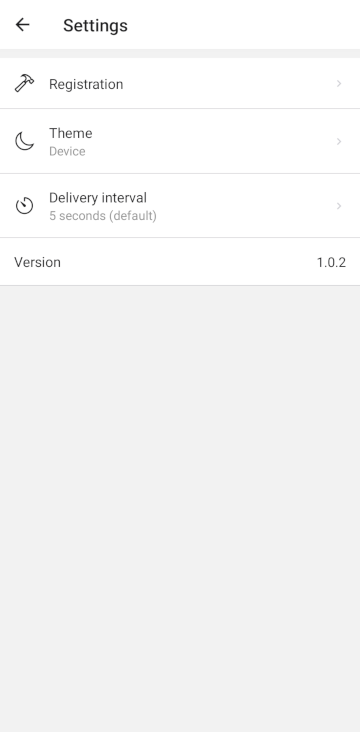The image is a screenshot of a mobile device's settings interface, likely an iPhone or iPad, given the layout and design consistency typical of Apple products. The background displays a monochromatic color scheme featuring shades of black, gray, white, and cream. At the top, a black header labeled 'Settings' with an arrow pointing left indicates the current section.

Directly beneath the header, several interactive sections are listed: 

1. **Registration**: Identified by a hammer icon.
2. **Theme**: Marked with a moon icon.
3. **Device Info**: Suggested by the context.
4. **Delivery Interval**: Accompanied by an icon resembling a timer set to 10 seconds before midnight. The default interval is set to 5 seconds.

To the right of each section title, light-colored arrows suggest that these items currently cannot be clicked for further options. At the bottom of this interface segment, the text 'Version 1.0.2' is displayed, indicating the software version.

All the detailed information occupies the upper half of the screenshot, while the lower half remains completely blank, reinforcing the focus on the available settings.